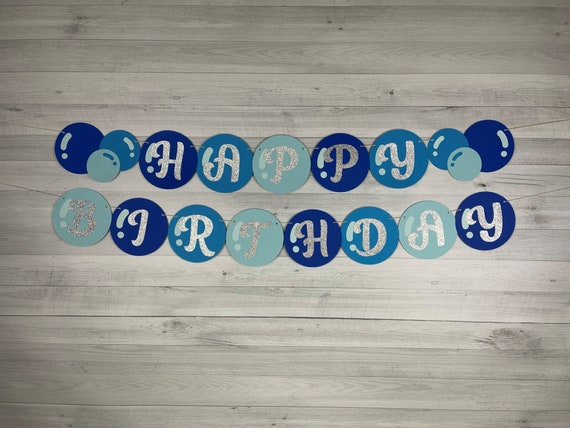This image captures a festive "Happy Birthday" decoration set against a light gray background with a wood grain design. Two banners, threaded on strings, are centrally arranged. Each banner is composed of balloons in a gradient of blue tones ranging from deep royal blue and indigo to turquoise and a lighter blue. The upper banner spells out "HAPPY," with one large, white, glittery letter on each balloon, progressing in color from darkest to lightest blue. The lower banner spells "BIRTHDAY" in a similar style and color transition.

Each balloon features delicate white markings and dots on the left side, artfully simulating light reflections. Additionally, the start and end of the "HAPPY" banner are accented with clusters of three balloons each, in varying sizes and blue shades. These clusters are not repeated on the "BIRTHDAY" banner below, which maintains a straightforward alignment of individually lettered balloons. The overall effect is a cohesive and visually appealing celebration banner designed to be suspended across a wall or between pillars.